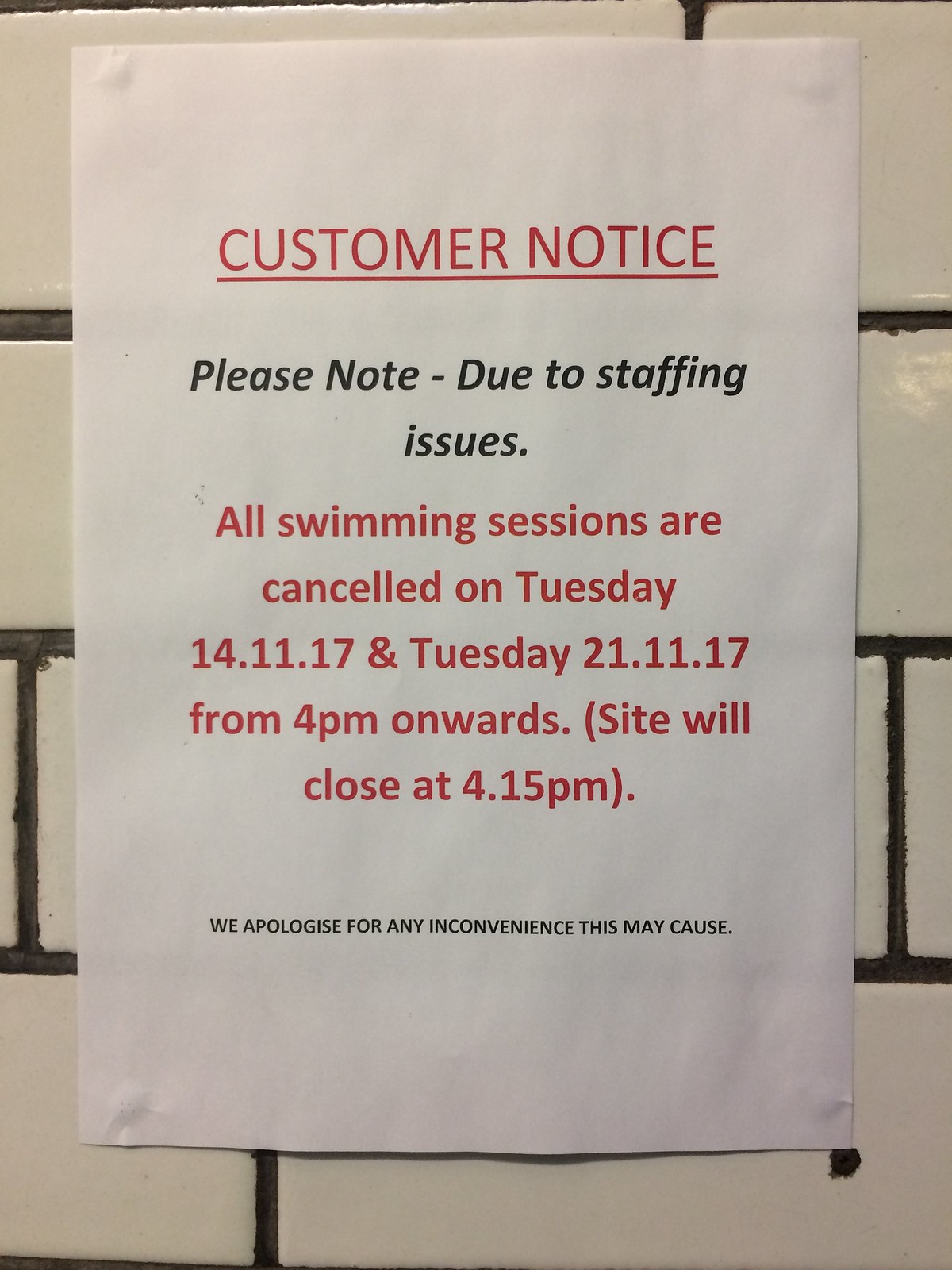The image depicts an indoor setting with a piece of white computer paper posted on a white tiled wall, characterized by long rectangular tiles with black grout, reminiscent of an old subway style. This rectangular notice, taller than it is wide, is taped centrally on the wall. The sign starts with a top-center heading in large red text that reads "Customer Notice," underlined in red. Below this, in black bold lettering, it states, "Please note - Due to staffing issues." Further down, in bold red print, it announces, "All swimming sessions are canceled on Tuesday, 14-11-17 and Tuesday, 21-11-17 from 4 p.m. onwards," with an additional note in red within parentheses, "Site will close at 4.15 p.m." Finally, at the bottom of the notice, in small black print, the sign reads, "We apologize for any inconvenience this may cause."